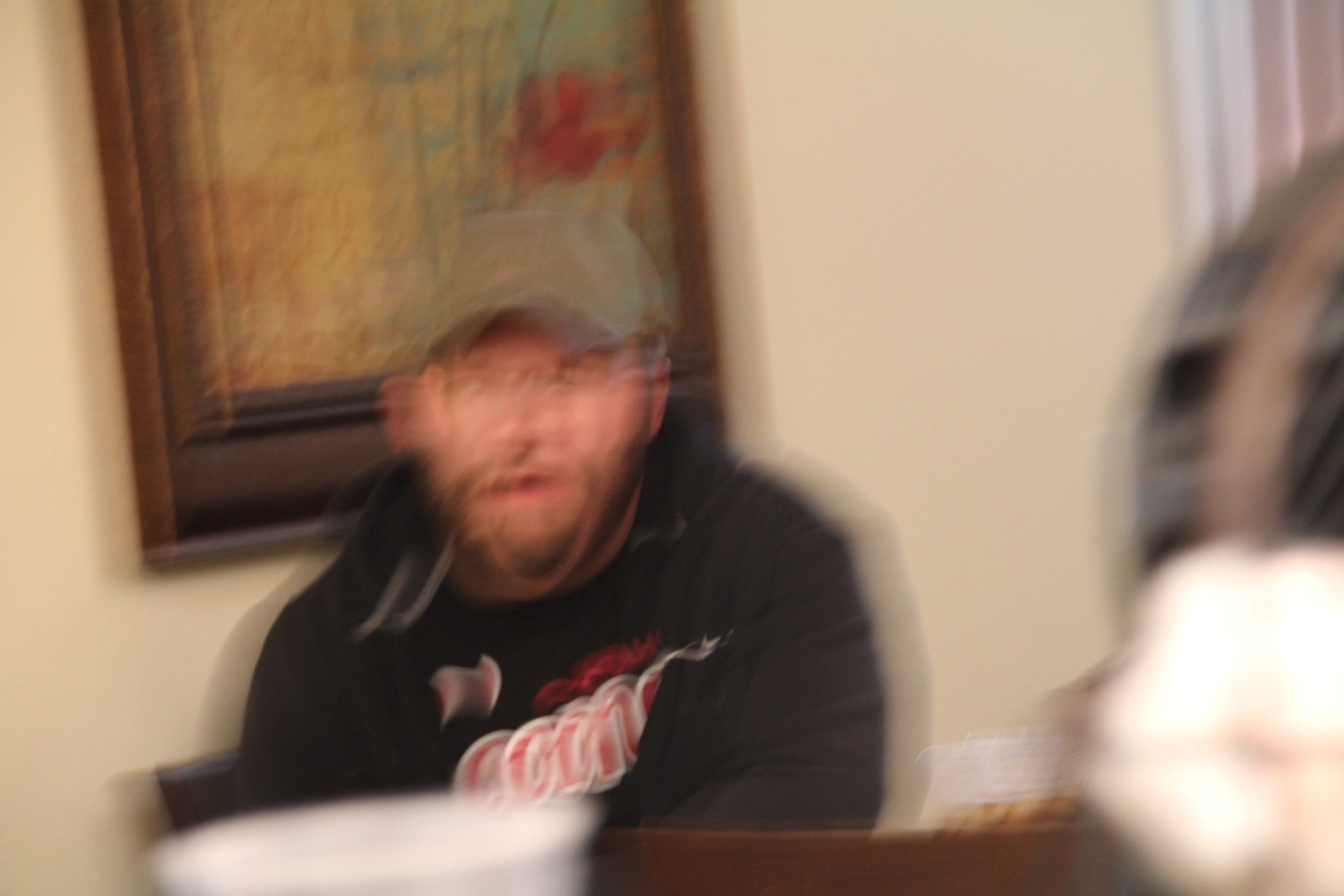This image, taken indoors in a dining area, is extremely blurry, suggesting the photographer moved the camera as the shutter closed. It captures a man seated at a table wearing a black jacket over a black t-shirt with red writing, paired with an olive green ball cap with a folded bill. There's a large framed piece of art behind him, encased in a thick brown wooden frame, featuring what seems to be a red flower on the right side of the print. The wall behind is a light off-white or cream color. The man appears to have a beard and mustache, and he is sitting in a brown wooden chair, part of which is visible on the left side. In the image's foreground, the top of a white plastic cup is visible, and on the bottom right, there's an indistinct, blurry outline of what might be a hand.